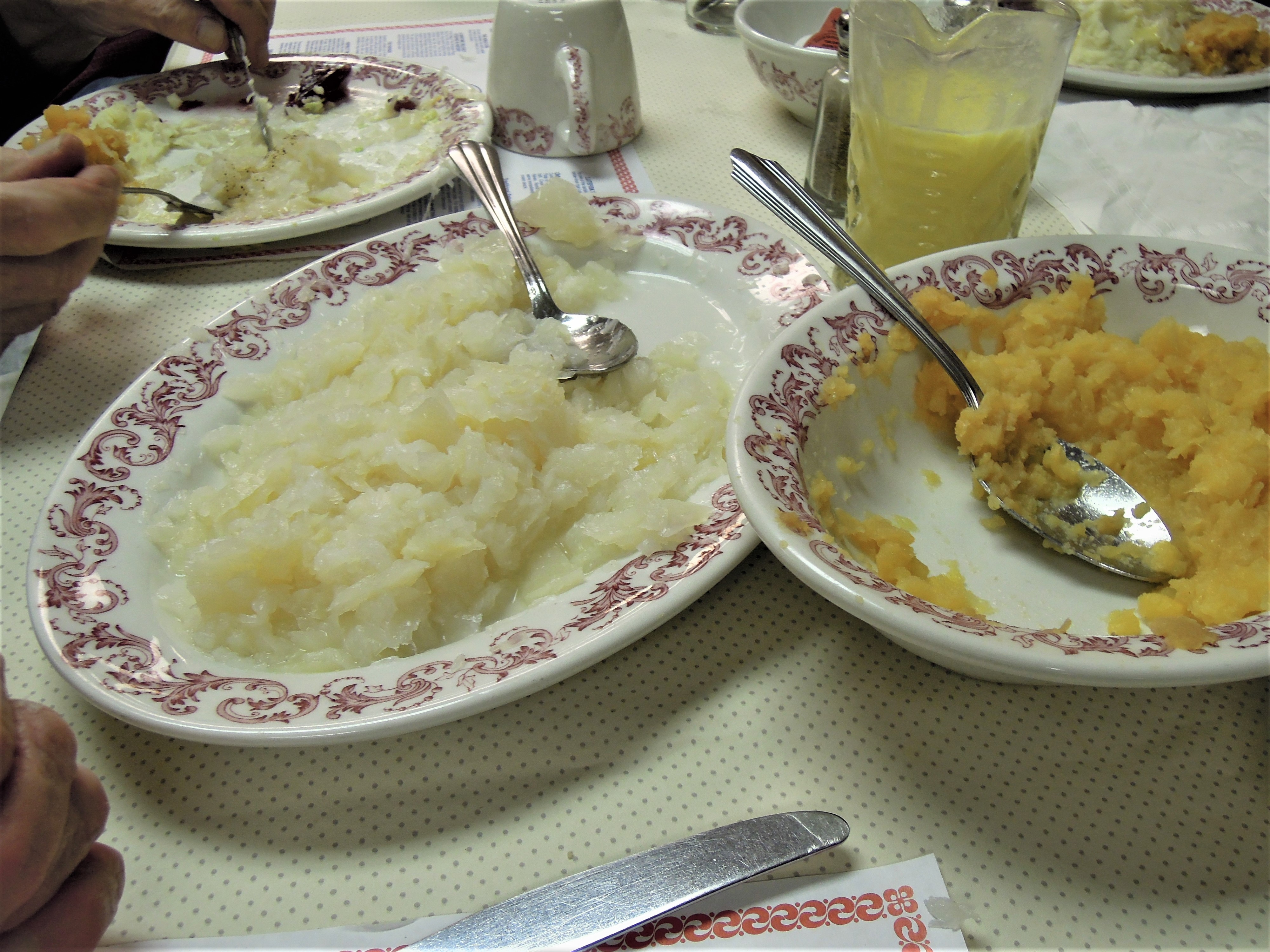The image shows a large, square picture of a dining table covered with a beige tablecloth adorned with small dotted patterns that resemble vents. At the upper left corner, two male hands hold a knife and fork, poised over a plate that contains what appears to be sauerkraut and possibly sweet potatoes or another starchy side. The table is set with white plates featuring red, swirling decorations along their borders. 

In the lower left corner, another hand is visible, holding a spoon over an oblong-shaped plate piled with a generous serving of sauerkraut. Adjacent to it, on the right, is a round plate with the same decorative pattern, holding what looks to be sweet potatoes, mashed squash, or a similar thick, starchy food. Both plates have shiny silver spoons, indicating they are relatively new.

In addition to the food, there's a clear glass pitcher filled with a yellow or dingy orange liquid, possibly lemonade or juice, placed near the plates. An overturned cup can be seen at the top of the image, adding a slight touch of casual disarray to the overall scene. Various utensils, including a visible butter knife at the bottom of the image, complete the detailed table setting.